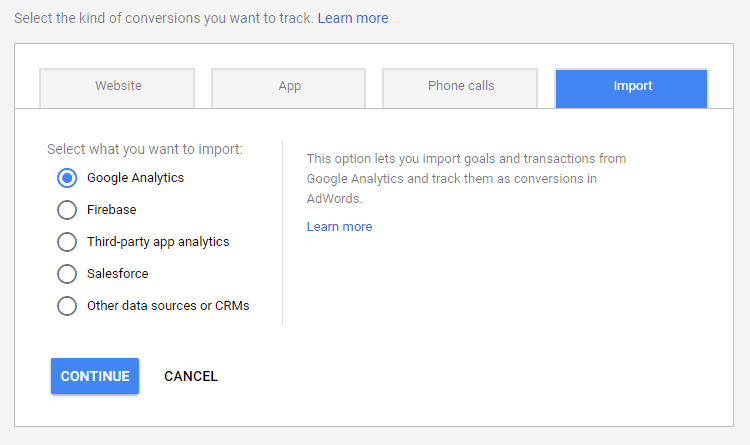A screenshot of the Google AdWords settings panel with a gray background and a large, centered white box. At the top left of the panel, a prompt in large gray font reads, "Select the kind of conversions you want to track," accompanied by a "Learn more" link in blue font to the right. Inside the white box, a horizontal row of tabs is displayed at the top, each indicating different conversion sources: "Website" in small gray letters, "App," "Phone calls," and on the far right, a blue "Import" tab with white lettering. Below these tabs, a section is labeled "Select what you want to import" on the left. This section features a vertical list of clickable options for importing data: Google Analytics (already selected), Firebase, third-party app analytics, Salesforce, and other data sources or CRMs. To the right of the selected Google Analytics option, an informational note explains, "This option lets you import goals and transactions from Google Analytics and track them as conversions in AdWords," with another "Learn more" link in small blue letters below. At the bottom left of the panel, a blue "Continue" button and a "Cancel" option in large black bold letters are available for action.